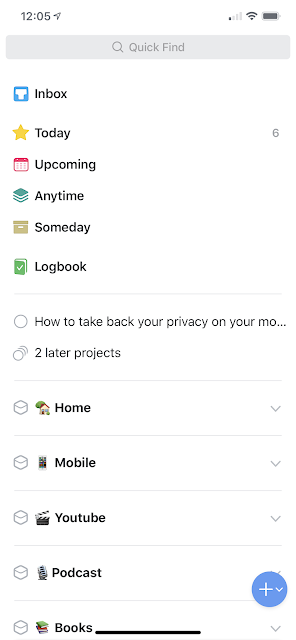This image is a screenshot of a mobile device home screen. At the top left corner, the time displayed is 12:05. Adjacent to the time are notification and location icons. On the top right corner, there is the network signal bar indicating 1 out of 4 bars in signal strength. Next to it, the Wi-Fi signal shows a full 3 out of 3 bars, and the battery level is fully charged.

Below this status bar is a search field featuring a magnifying glass icon and the placeholder text "Quick Find." The screen also displays several categories and items: "Text to Your Inbox," "Today," "6," "Upcoming," "Anytime," "Some Day," "Logbook," "Home," "Mobile," "YouTube," "Podcast," and "Books." Additionally, there is a noted section or title reading "How to Take Back Your Privacy on Your Soolator Projects."